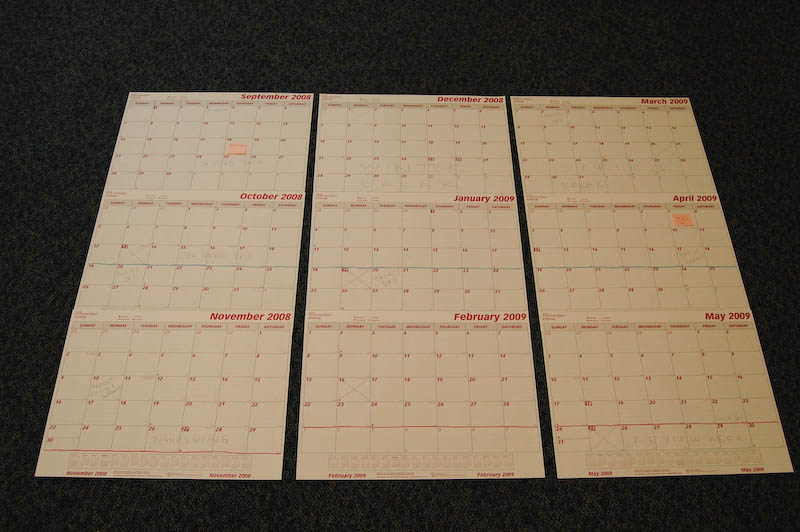This image depicts nine pages from a calendar, precisely arranged in a three-by-three grid on a dark grey, carpeted floor. From top to bottom and left to right, the calendar pages display the months as follows: September 2008, October 2008, November 2008 in the first row; December 2008, January 2009, February 2009 in the second row; and March 2009, April 2009, May 2009 in the third row. Each calendar page is white with dates and text printed in red ink, featuring a grid layout where the dates are positioned in the top left corner of each cell. Some of the pages have writing or markings like X's across certain days, although the specific content is not legible.